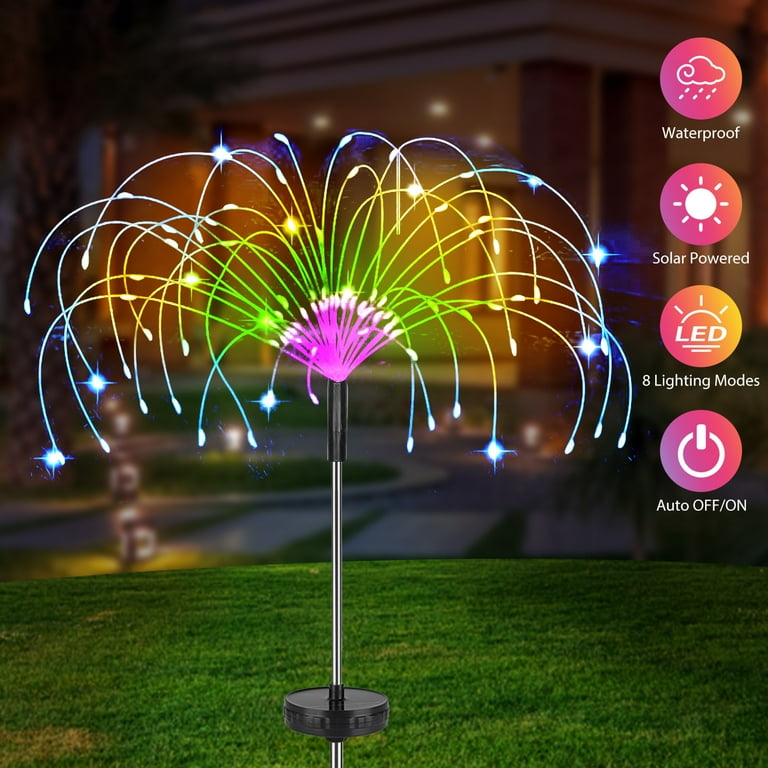The image depicts an animated illustration of an outdoor LED lighting fixture set against what appears to be a well-manicured lawn. Central to the image is a metallic pole with black tips and a base resembling a chopped-off plunger. Emanating from a black cylinder near the top of the pole are multiple light strands, arching outward like the leaves of a palm tree or the spray from a sprinkler system. The lights transition in color from pink at the base to green, then yellow, and finally blue at the tips. The background includes a partial glimpse of a governmental or landmarked building. On the right side of the image, there are four pink circles with white symbols and text: the top circle shows a rain cloud with the label "waterproof," the next a sun denoting "solar powered," followed by a circle indicating "8 LED lighting modes," and the last displays a power symbol with the label "auto on/off." This suggests that the light offers versatile, weatherproof, and energy-efficient functionality suitable for outdoor use.